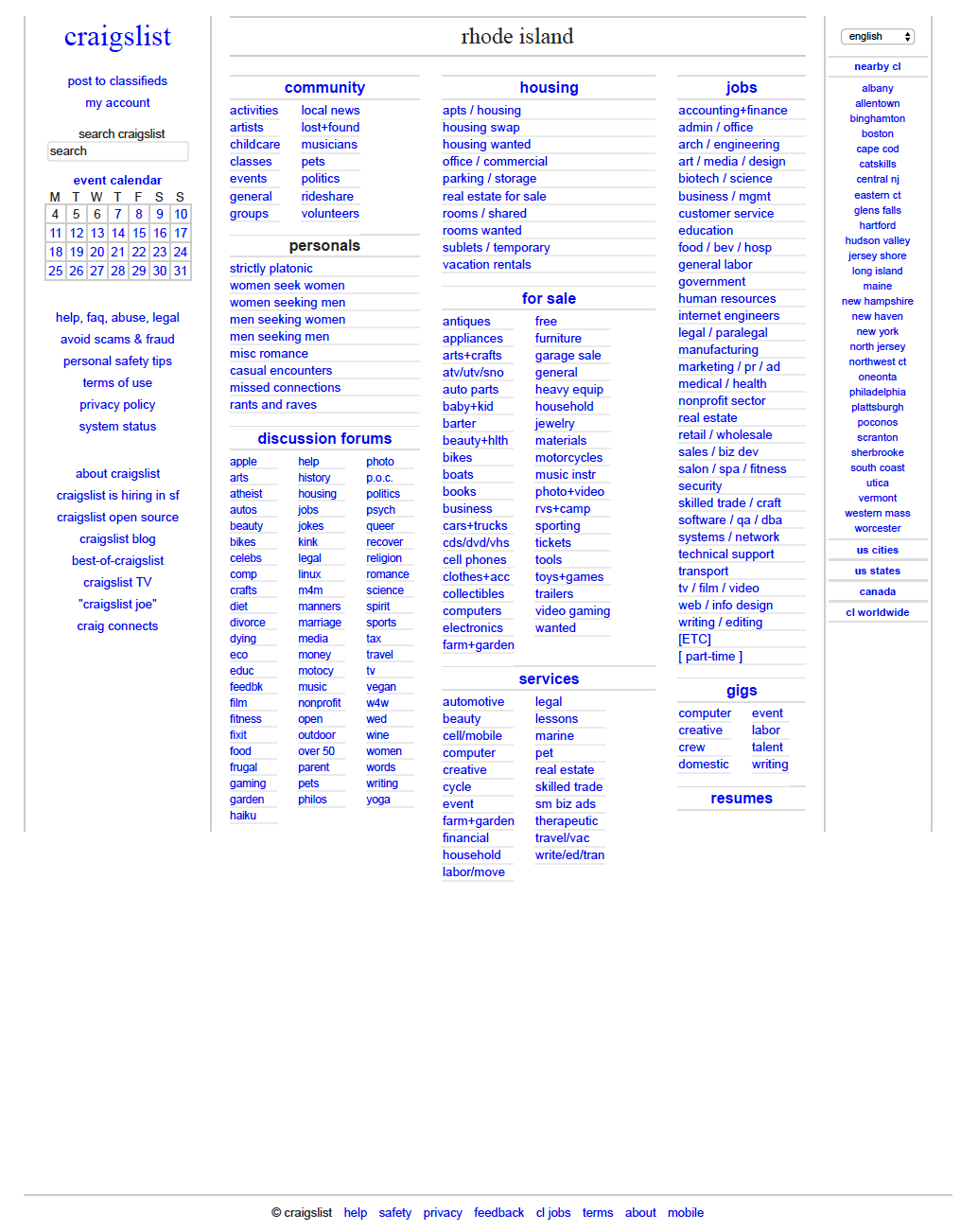Screenshot of Rhode Island Craigslist Page

The image showcases a screenshot of a Rhode Island Craigslist page with a predominantly white background. At the very bottom, there is a thin gray horizontal line. Below this line, the word "Craigslist" appears on the left in black, flanked by a copyright symbol. Adjacent to this, various options are listed in blue: help, safety, privacy, feedback, CL jobs, terms, about, and mobile.

On the left-hand side of the image, a vertical navigation bar is visible. At the top, it says "Craigslist," followed by options to post classifieds, access my account, and a search Craigslist option accompanied by a search bar. Below this, there is a calendar, followed by numerous listing categories including Help, FAQ, abuse legal, avoid scams and fraud, personal safety tips, terms of use, privacy policy, system status, about Craigslist, Craigslist is hiring in SF, Craigslist open source, Craigslist blog, best of Craigslist, Craigslist TV, "Craigslist Joe," and Craig Connects.

The central section confirms that this page is for Rhode Island. Different categories are displayed, such as community, housing, jobs, and personals—with 'personals' highlighted in black while others are in blue. Additional categories listed include for sale, discussion forums, services, gigs, and resumes.

On the right-hand side, another column presents nearby Craigslist options for different locations.